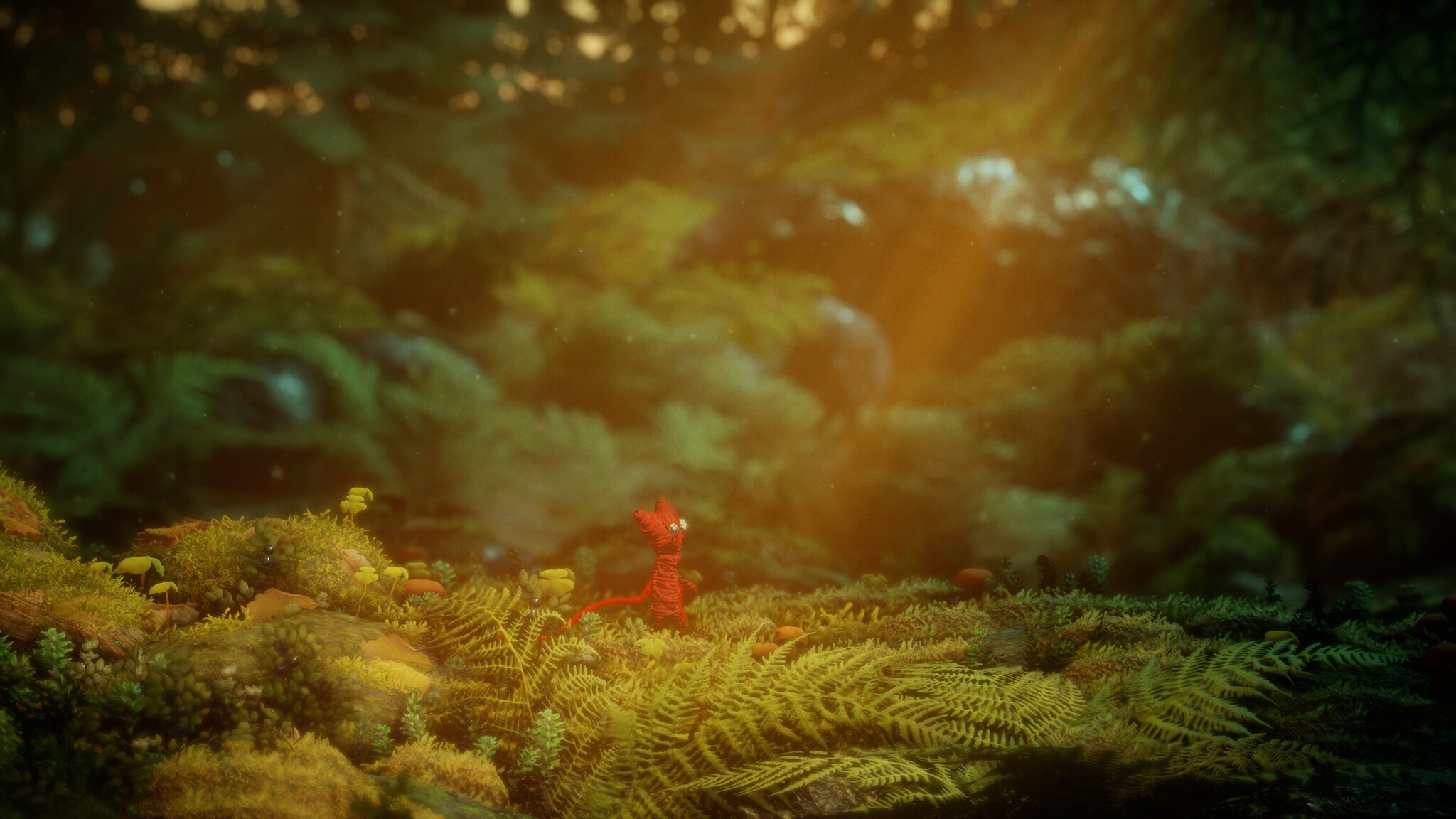This digital illustration presents a detailed forest floor scene teeming with life. The ground is covered with an array of small brown rocks and patches of vibrant green moss. Tiny plants emerge intermittently amidst the undergrowth, their leaves appearing fuzzy and elongated, reminiscent of delicate fern fronds. Nestled among these ground elements, you can see densely packed foliage, including lush green plants and thick bushes. Sunlight filters through the canopy above, casting a warm glow over the scene and adding depth to the various shades of green. In the blurred background, a gray shape is faintly visible, possibly a rock partially obscured by the surrounding vegetation. Adding a touch of whimsy and intrigue, a small red creature is nestled among the flora, standing out vividly against the natural palette of the forest floor.